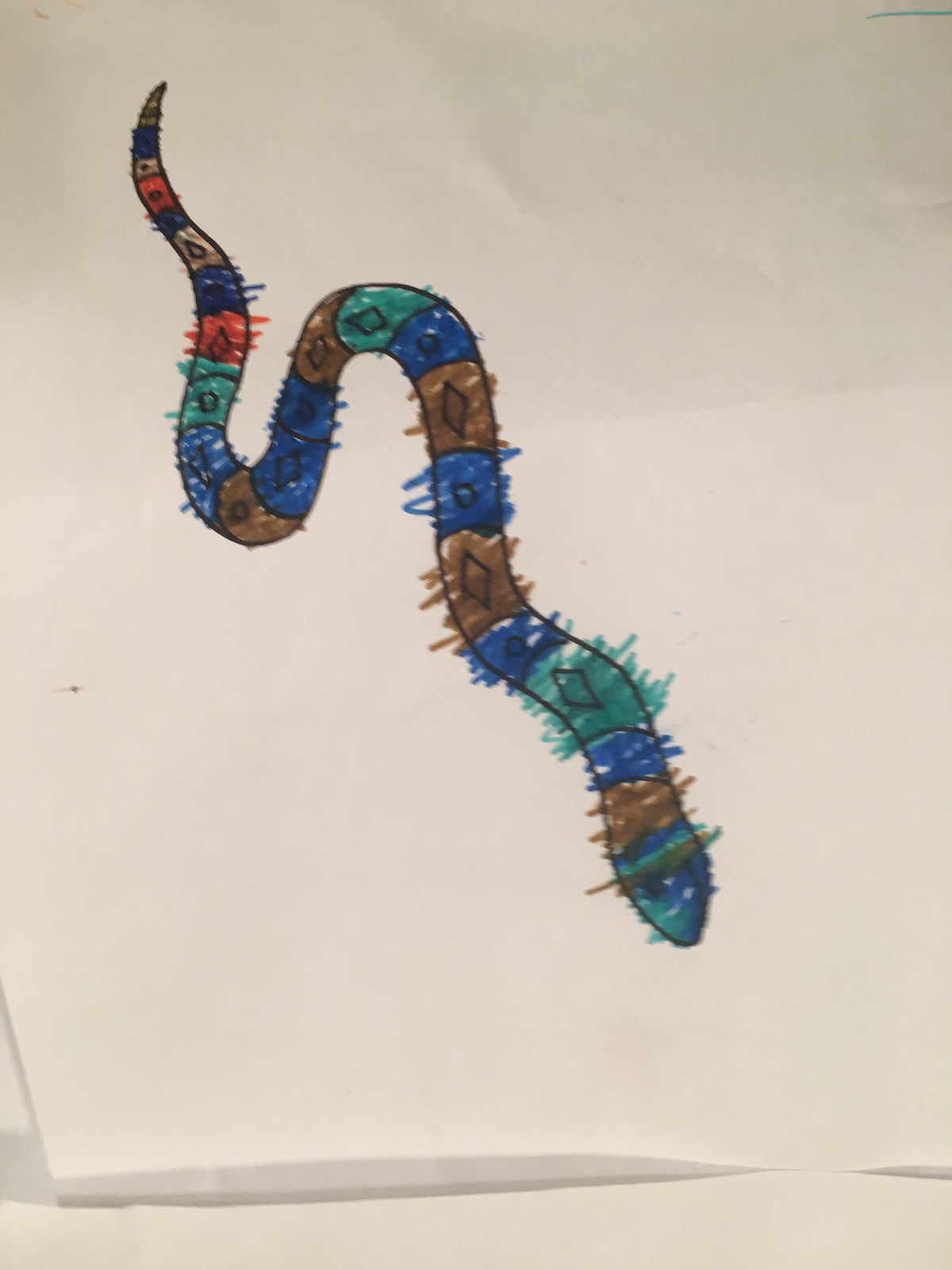This image showcases a vividly colored-in coloring page of a snake, meticulously completed using markers. The snake, captured in a black outline, slithers gracefully across the white paper with a sinuous, curvaceous form. Its body is cleverly divided into small, individual squares, each containing the outline of a diamond, creating a striking geometric pattern. As the snake's body tapers towards the pointed tip of its tail, the variations in color become particularly pronounced. Each square along its length is filled with a distinct shade, predominantly featuring hues of green, brown, and blue, interspersed with two vibrant orange squares that add a splash of unexpected color to the composition. The detailed coloring and precise line work make this snake illustration a captivating and intricate piece.